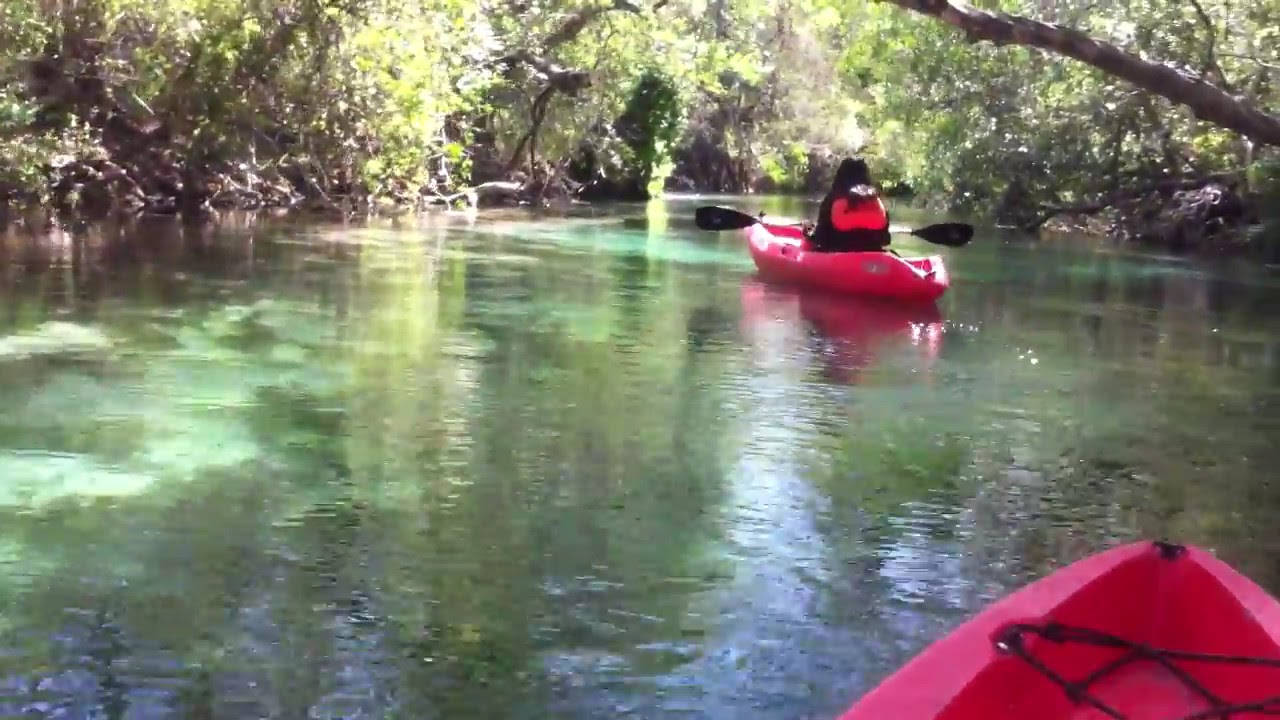In this image, a serene river scene is captured from the perspective of someone seated in a red canoe. The canoe's tip, along with a black wire, is visible in the bottom right corner of the frame. The calm, green-tinted waters subtly reflect the dappled sunlight filtering through a dense canopy of trees that arch over the river. The scene is enriched with various shades of green and hints of yellow, brown, and white from the surrounding foliage. Towards the top center of the image, another red canoe can be seen, with a woman wearing a red life vest and holding black paddles. The woman appears to be rowing the canoe gently through the tranquil waters. The riverbanks are lush with verdant vegetation, including branching tree trunks and roots extending into the water, adding to the sense of immersion in this secluded, natural setting. The photograph, taken in the middle of the day, highlights the vibrant colors and peaceful atmosphere of the outdoors.